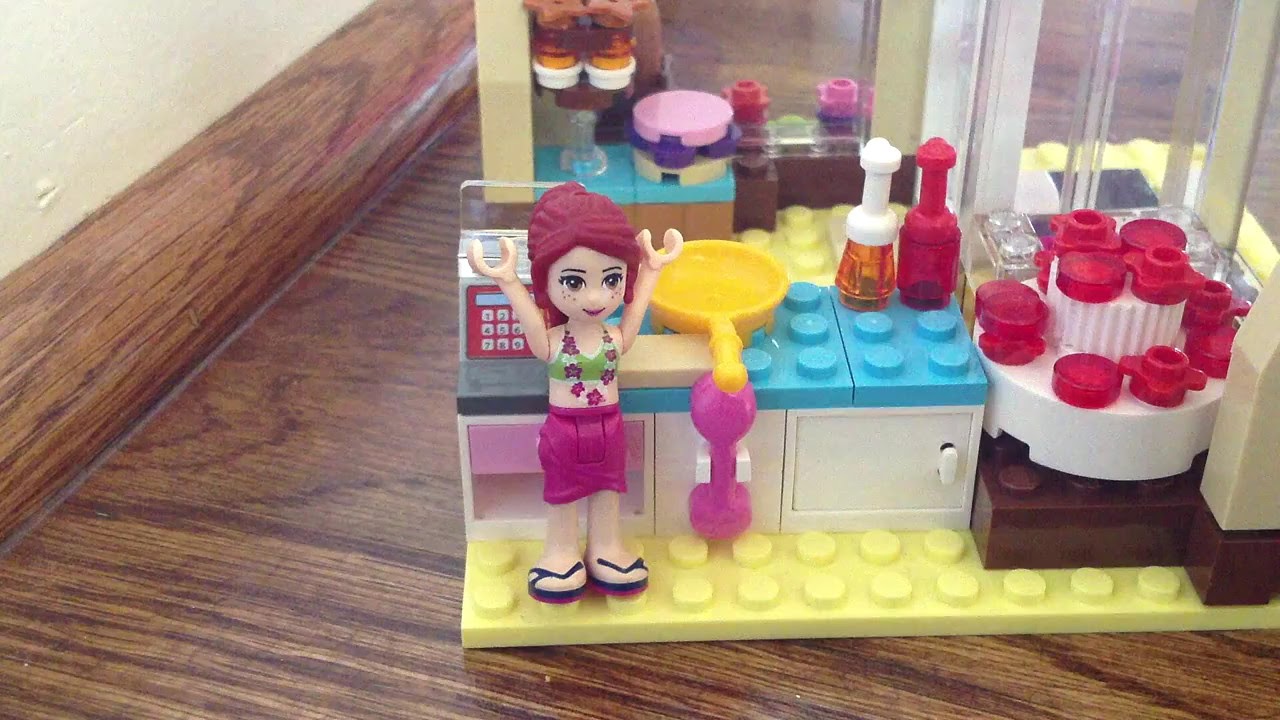This photograph showcases an intricately built Lego diorama depicting a fully equipped kitchen, set against a brown wooden floor. The floor's warm tones contrast with the vibrant colors of the Lego pieces used in the kitchen. The main focus is a Lego female character standing in the kitchen with her arms raised. She has striking raspberry red hair tied back, freckles, and is dressed in a green bikini top adorned with a floral pattern, magenta skirt or shorts, and blue sandals.

In the background, behind the female figure, there's a cooktop featuring a bright yellow frying pan. The right side of the kitchen includes a blue countertop with white cabinetry below, flanked by a keypad and what looks to be a cash register or a microwave. Additional kitchen utensils and food items are scattered around, including cups, plates, a mixer, ketchup and mustard bottles, and a cake resembling white blocks with red accents. 

The floor of the miniature kitchen itself is composed of yellow Lego blocks, enhancing the overall bright and playful ambiance of the scene. The setup is bordered on the left by brown railings and a cream-colored wall, which subtly frame the cheerful Lego kitchen.